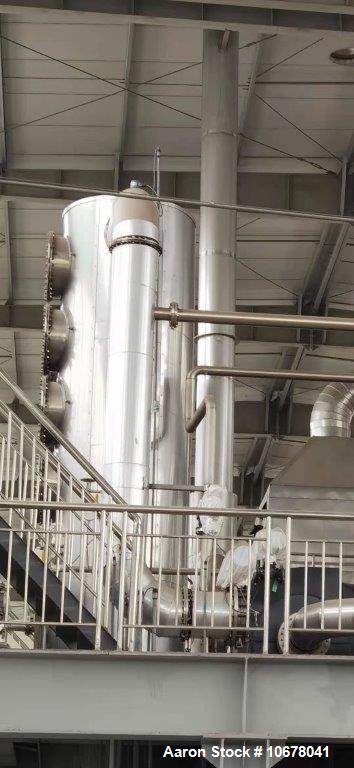The image depicts an interior view of a factory, featuring a complex arrangement of industrial machinery and structural elements. Central to the image is a large silver cylindrical tank with several dark-colored round extensions resembling valves, likely designed for connecting pipes. This tank is prominently positioned, with a significant pipe running through its middle and extending upward, suggesting a possible transportation of liquid or gas. Surrounding the tank are other pipes of similar dark metal color, which intertwine and connect to various parts of the factory.

In the foreground, there is a silver metal railing composed of horizontal and vertical bars, providing a barrier along a walkway. To the left of this railing, a set of stairs ascends diagonally, adding to the multi-level structure of the factory. The flooring beneath the walkway appears to be a metal platform, and an identifier with "AIR" and stock number "10678041" is visible in this area, likely referring to the photo details.

The factory ceiling is supported by large steel beams with horizontal lines sectioning it into compartments, maintaining the industrial aesthetic. A long round rod-like beam, with visible grooves, extends from the ground to the ceiling. Additionally, there are metal parts, possibly clamps or connectors, aligned along the upper portion of the image, contributing to the intricate network of support structures.

Overall, the image captures the robust and utilitarian design of a factory interior, highlighting the integration of heavy machinery with structural supports and pathways.